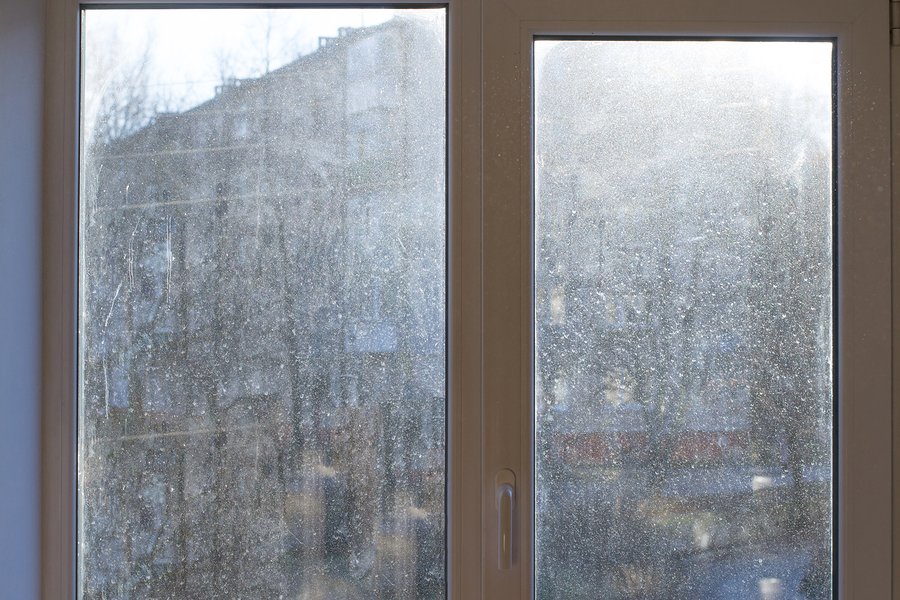This color photograph features a set of two sliding glass doors or possibly European-style windows, both equipped with brown frames and downward-pointing brown handles that suggest they could be turned to open. The doors or windows are notably grimy, with sun shining from the top right corner, illuminating the accumulated dirt, dust, and rain streaks. Through the cloudy glass, faint outlines of an apartment building and nearby trees can be discerned. The wall to the left is painted a dull light blue. No people, animals, or writing are present in the image, and the setting of the photograph remains unspecified.